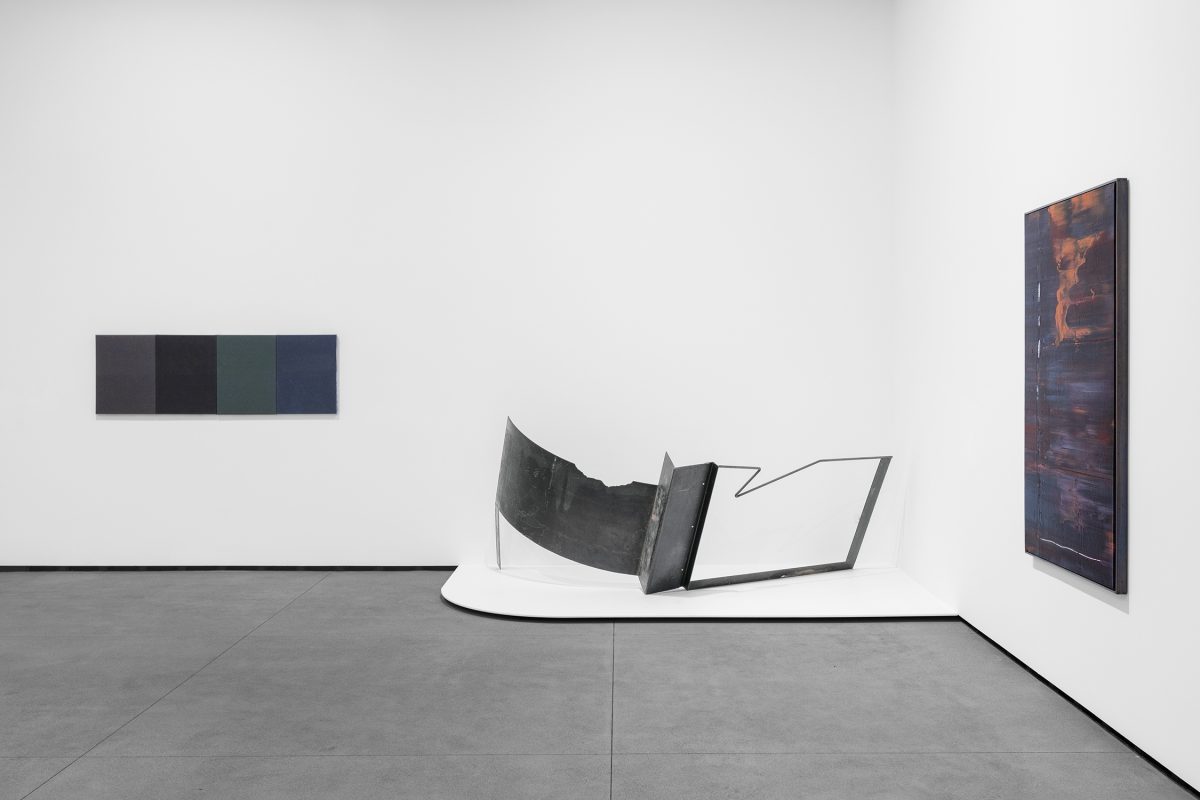The image depicts a meticulously designed architectural illustration of an art exhibit within a museum. The room features distinctly large, dark gray ceramic tiles forming the floor, which transitions through a straight line into a half curve leading back to a wall. The walls are tall and immaculately white, enhancing the room's modern aesthetic and creating a perfect backdrop for the artwork on display.

On the right side, a curved wall is hinted at by an unusual painting that appears to carry over the invisible curve due to its artistic depiction, although parts of it show signs of chipping. Adjacent to this, on the same right wall, hangs another framed painting that showcases a striking contrast of bronze, black, and touches of white, notable for its vertical elongation and dramatic use of dark tones layered in sweeping brushstrokes.

On the farthest left wall, an abstract rectangular composition splits into four distinct color blocks—dark gray, black, navy green, and dark blue—providing a visually captivating geometric display. Additionally, in the main visual space, an intricate metal sculpture draws attention; it is a rectangular piece of dark gray metal juxtaposed with what appears to be a glass element connected by wire, evoking a powerful, almost shrapnel-like quality.

The precision of the room’s layout, the harmonious play of colors, and the diversity of the art pieces collectively create a compelling and cohesive museum exhibit designed to immerse visitors in a thought-provoking artistic environment.